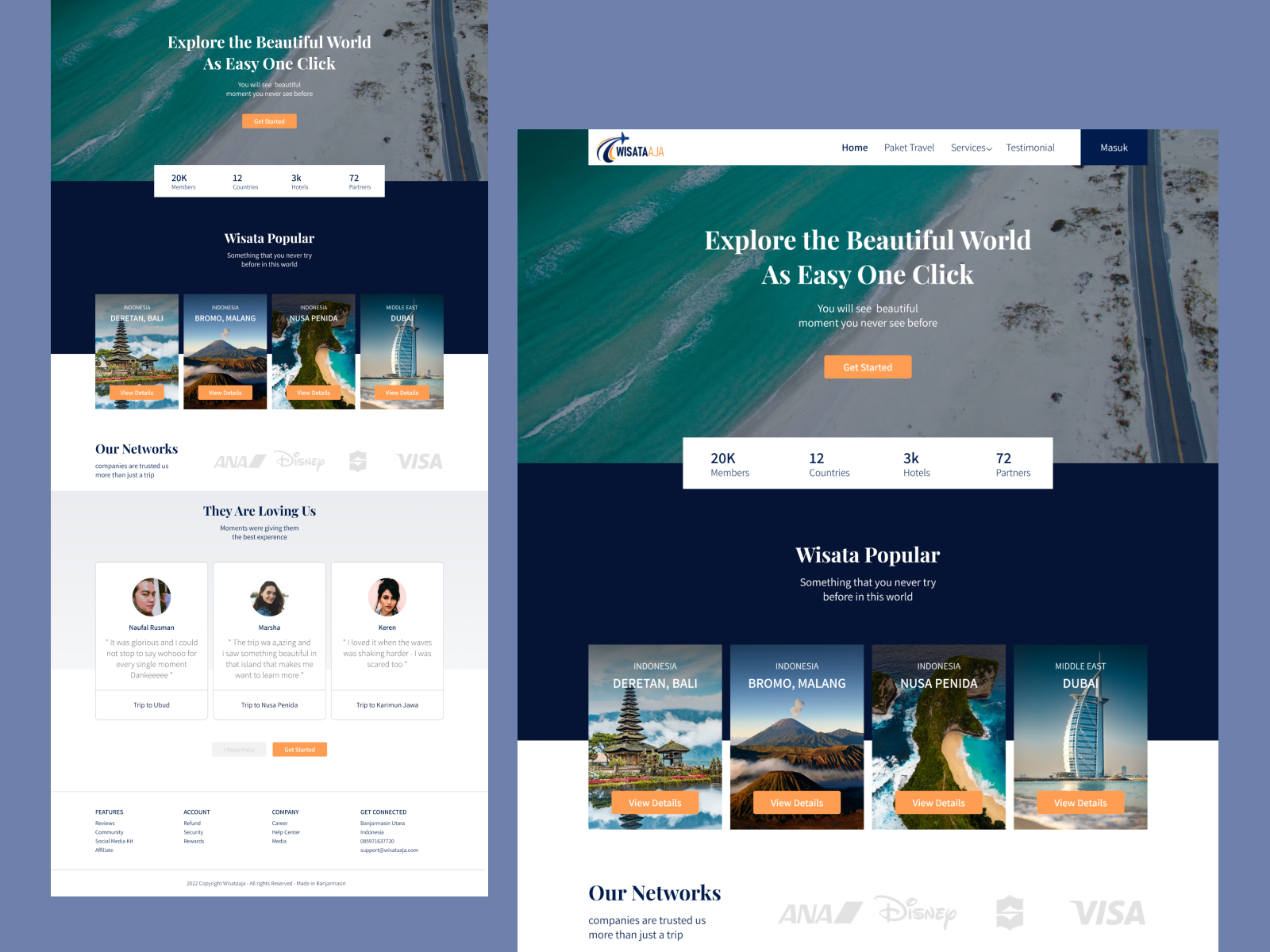This image is a screenshot from Wisata, a vacation booking website, showcasing both its mobile and desktop versions. The striking feature of both versions is the stunning background image of a beautiful beach with aqua teal water captured from an aerial view. The beach showcases pristine white sand intersected by a road cutting through it.

Despite the text being quite small, you can make out some of the key details. The company’s name, Wisata, is prominently displayed along with the tagline: "Explore the Beautiful World is Easy. One click." The message assures users that they will experience "a beautiful moment you never see before." The interface invites users to get started and highlights impressive statistics, including 20,000 members across 12 countries, 33,000 hotels, and 72 partners. Popular destination options showcased on the site include Bali and Dubai.